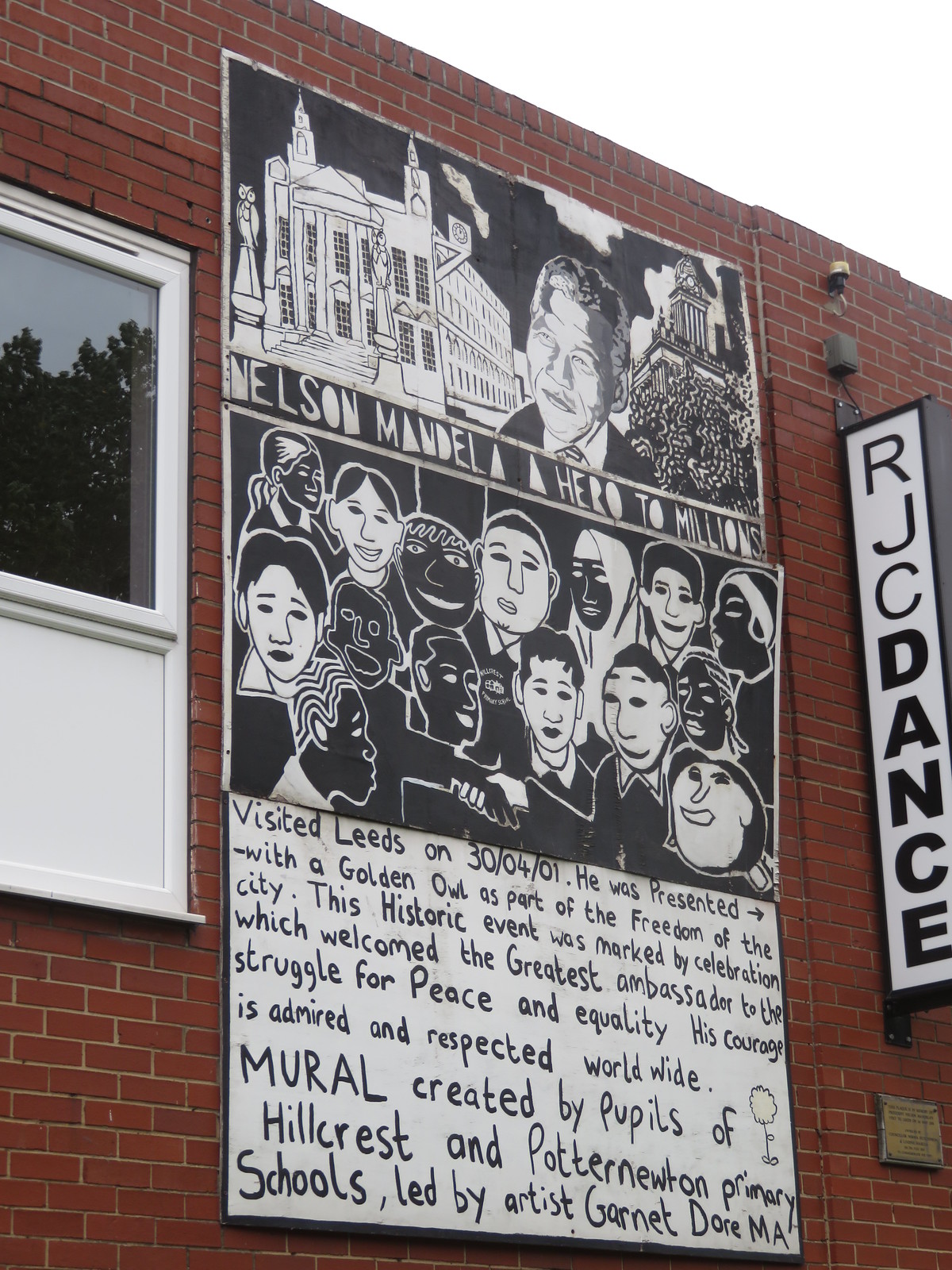This portrait-oriented photograph captures a striking mural painted on the red brick wall of a two-story building. The mural, black and white in color and divided into horizontal thirds, pays homage to Nelson Mandela. To the left of the mural, a white-framed window is visible, while to the right, a white sign with bold black letters reads "RJC Dance."

At the top section of the mural, white text on a black background reads "Nelson Mandela, a hero to millions." The centerpiece of this section features a graphic drawing of Nelson Mandela, flanked by two buildings—a white structure on the left and another building with figures standing underneath on the right. In the middle section, a diverse group of people is depicted, their black and white faces symbolizing unity, with two individuals of opposite colors shaking hands at the center.

The bottom third contains text describing an important event: "Visited Leeds on 30/04/01. He was presented with a golden owl as part of the freedom of the city. This historic event was marked by a celebration which welcomed the greatest ambassador to the struggle for peace and equality. His courage is admired and respected worldwide."

The mural was created by pupils of Hillcrest and Potter Newton Primary Schools, under the guidance of artist Garnet Dory, M.A.